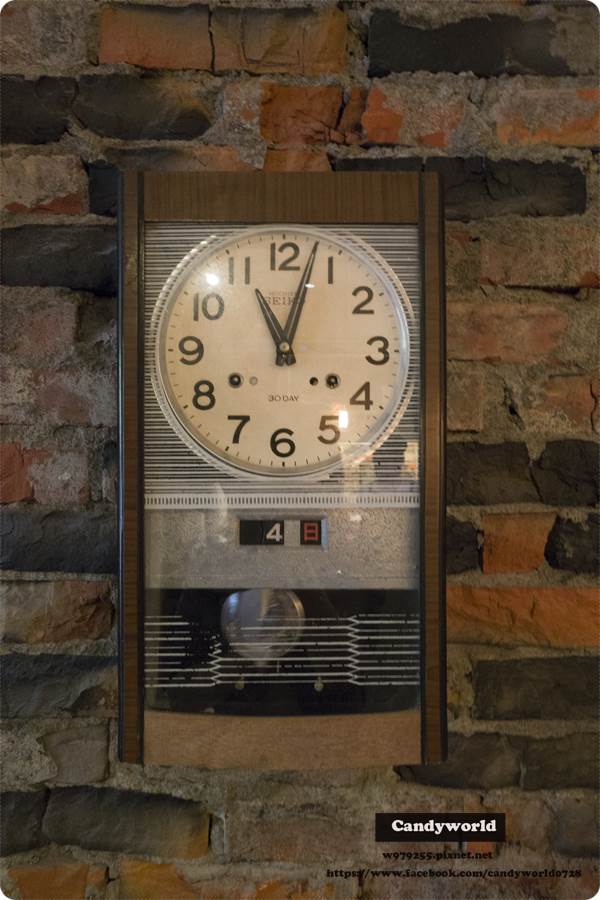This image features a vintage Seiko rectangular clock, likely from the 1980s or 1990s, prominently displayed against a rustic brick wall. The clock is set to 11:11 and intriguingly bears the brand name "Joday" as well, which may indicate a collaborative or lesser-known model. At the bottom of the clock, a digital display shows the number 48, though its significance is unclear. The clock itself boasts a decorative design, adding a touch of retro elegance to its environment. Additionally, a small logo at the bottom of the photograph reads "Candy Wall," possibly indicating a brand or artistic label.